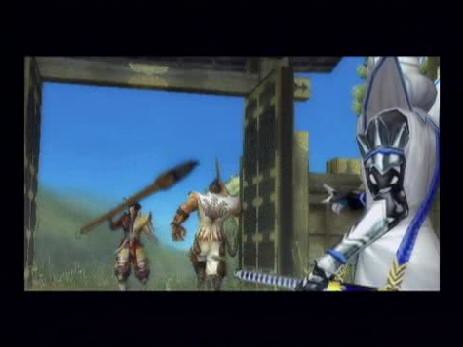A photograph captures a screenshot from a video game, likely taken with a camera aimed at a television or computer monitor. The scene appears dark, surrounded by the black borders of the monitor or TV in a dimly lit room. The screen displays a high-quality in-game cinematic or an animated movie scene, notable for the absence of gaming HUD elements.

On the right side of the image, a character clad in detailed white fantasy armor, accented with black on their left sleeve, commands attention. They wield an imposing serrated sword. The character stands within an open-air wooden pavilion, its door ajar, allowing a glimpse of a chaotic battle outside. Through the doorway, soldiers can be seen charging forward, one prominently holding a giant spear, contributing to the dynamic and intense atmosphere of the scene.